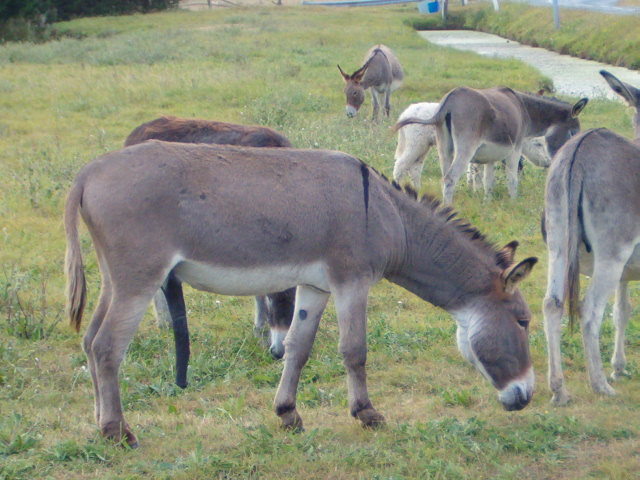This slightly underexposed, slightly blurry outdoor photograph was taken on a cloudy day and depicts a group of mules grazing in a field. The central focus is a light brown mule with a white belly and white face markings, looking down and to the right. Positioned directly behind it is another mule, partially obscured, with just its back and head visible. To the right, fading into the background, are four more mules. The field itself is composed of dry, yellow-green brushy grass interspersed with some dirt patches. There's a sidewalk or pavement area running from the top right-hand corner toward the center top of the image, accompanied by a light blue fence. In the backdrop of the image, darker green forest trees contrast against the grass. The mules, with their grey and brown fur, have distinctive white markings on their bodies, legs, and noses. Their tails hang down to the left, with some of them displaying dark-tipped black hair on their backs.